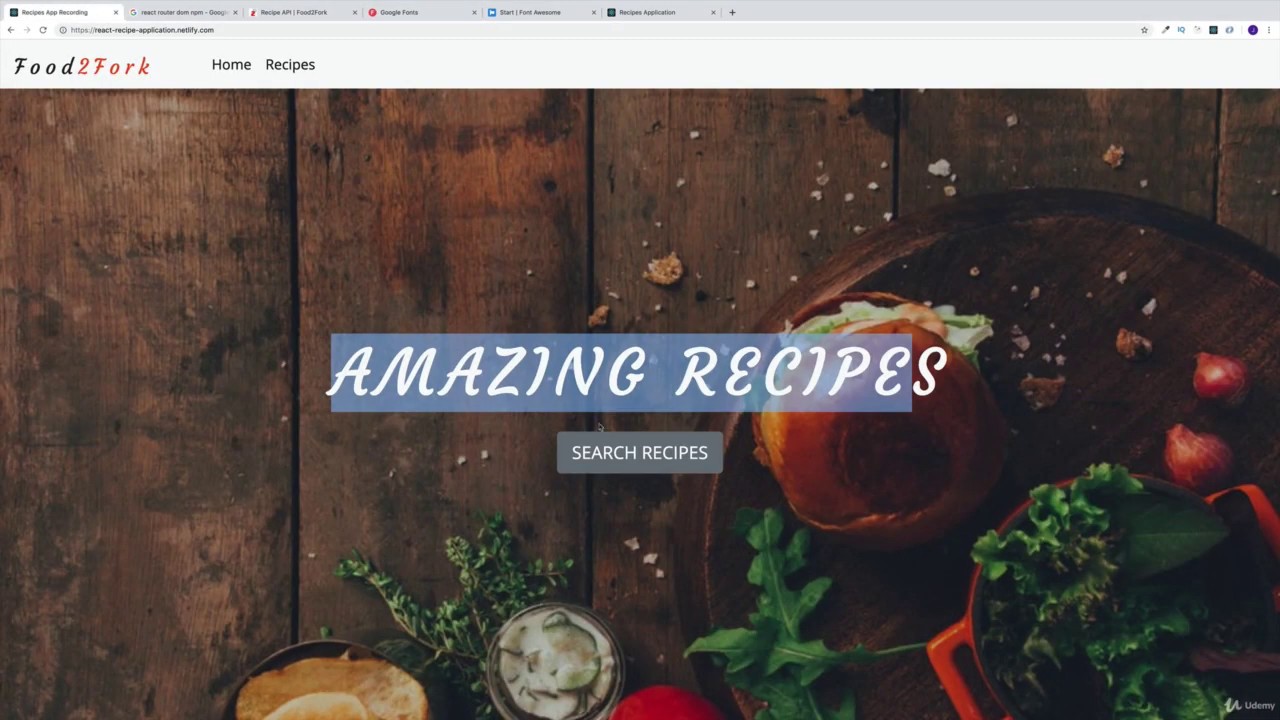This image is a screenshot of someone's desktop, featuring six open browser tabs, though the details of these tabs, including the URLs and titles, are too small to decipher. The active tab displays a web page titled "Food To Fork," with a logo employing an intriguing typographic design: the word "Food" is in black, followed by the number "2" in orange, which seamlessly transitions into "Fork," also in orange, making it appear as one continuous word. To the right of the logo, navigation options for 'Home' or 'Recipes' are visible, likely functioning as links to respective pages.

Beneath this header image is a top-down photograph of food, set on a polished dark brown wooden table. The centerpiece of the photo is a hearty sandwich or burger, identifiable by a well-toasted, thick hamburger or possibly a pretzel bun, with visible fillings that include some sort of meat and lettuce, though the exact type of sandwich remains unclear. The scene has a slightly messy charm, with crumbs and bits of food scattered around. Surrounding the sandwich are bowls containing various condiments.

Overlaying this image, the text "Amazing Recipes" is prominently typed, with part of it appearing to be highlighted, suggesting that the user might be in the process of editing the site. Beneath this text, there is a search bar labeled "Search Recipes," indicating the page's functionality for users to look up recipes. Overall, the image captures a moment of web design in progress, emphasizing a culinary theme.